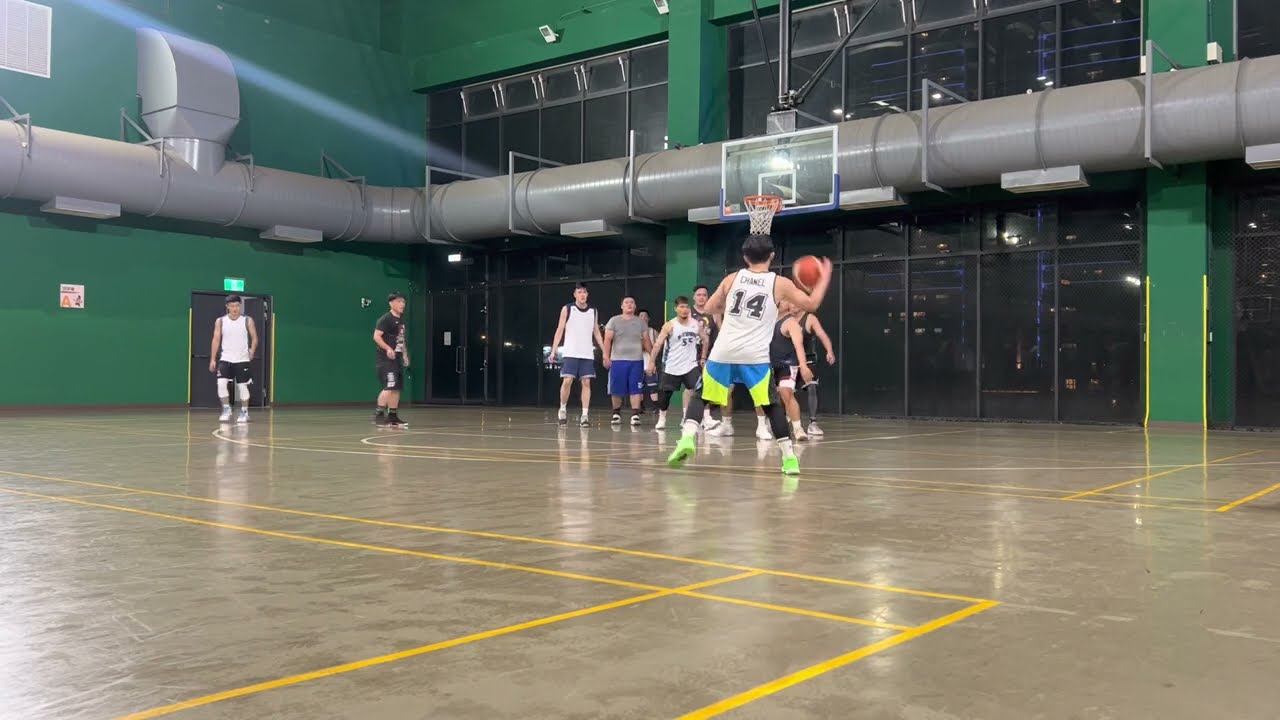The photograph captures a dynamic scene on a high school basketball court where a group of teenagers, possibly mid to late teens, are engaged in an intense game. The focal point is a player in the center, dribbling the basketball. This player, with his back to the camera, is distinguishable by his white jersey bearing the number 14 in blue, vibrant blue and green shorts, and eye-catching fluorescent green sneakers. The gymnasium is spacious and features a mix of components: large green columns and walls, a network of large gray metal pipes likely serving as a heating system, and a background that includes a basketball hoop mounted on these pipes. The court itself is a brownish hue with prominently marked yellow lines. Surrounding the main player are other participants, some in black jerseys, others in white, and one in a gray t-shirt, with most sporting dark-colored shorts. On the left side stands a man entirely in black attire—black t-shirt and black shorts—positioned next to another player in a white jersey with black pants, white leggings, and gray sneakers. Additionally, the background features a hint of windows and doors, and an unreadable sign is located on the left side of the photo, alongside visible numbers 55 and 14 on two of the players' jerseys.